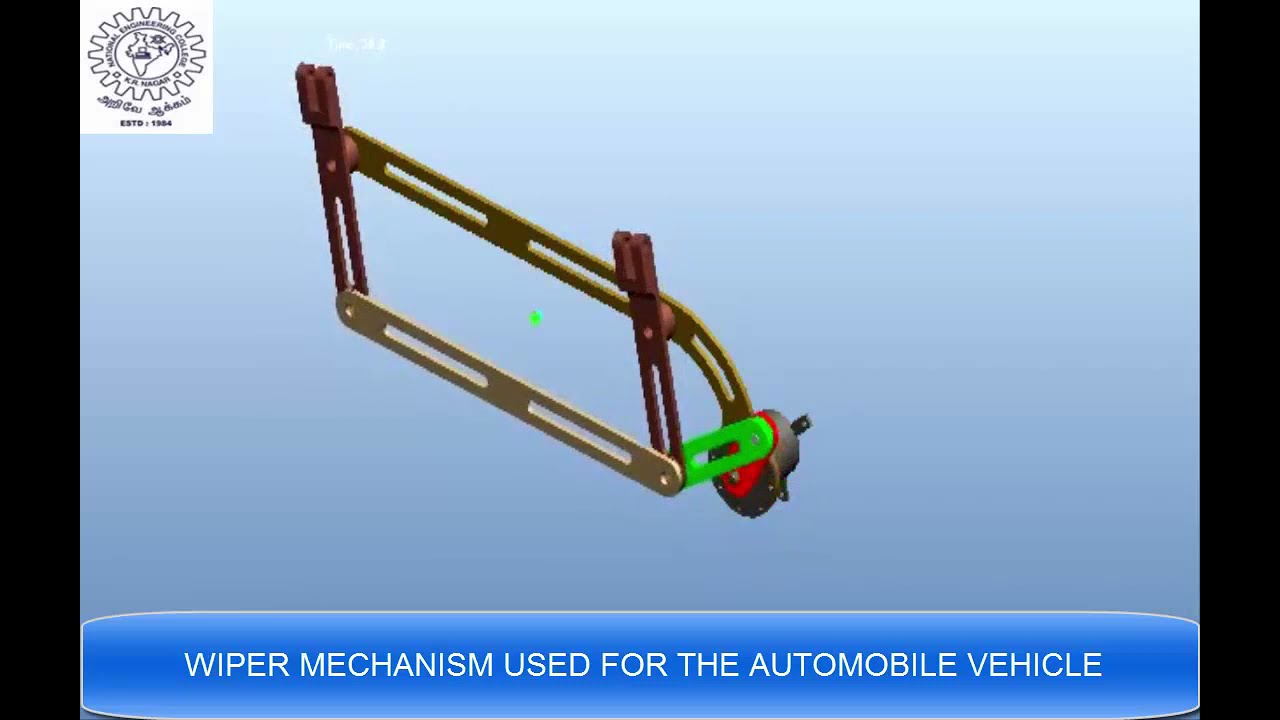The image features a wiper mechanism designed for an automobile vehicle, prominently displayed against a light blue background with black borders on the left and right sides. The device itself appears as a gold, rectangular mechanical arm, adorned with vertical maroon and horizontal gold posts. A notable green lever is attached to a red or orange head towards the lower right part of the mechanism, complemented by a neon green dot in the center. At the top left corner of the image, a black and white logo resembling a gear with a world map inside can be seen, accompanied by the text "Established 1994." The bottom of the image showcases a blue banner running from one black border to the other, with the phrase "WIPER MECHANISM USED FOR THE AUTOMOBILE VEHICLE" inscribed in large white capital letters, further outlined in white at the top and sides of the banner.